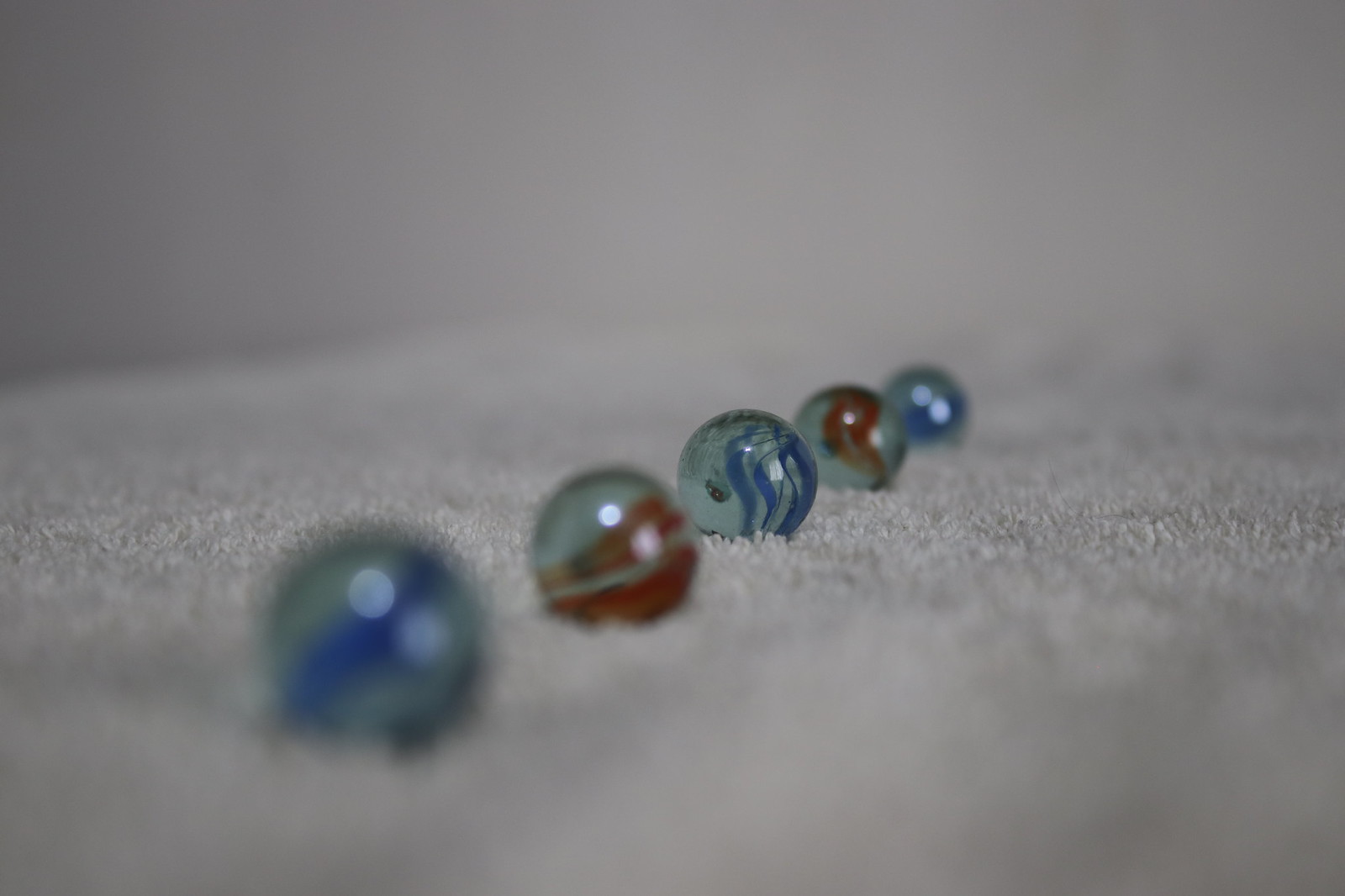The photograph showcases a neat row of five marbles arranged diagonally from the bottom left corner to the top right corner on a soft, fine-gray carpet. The focus is sharply on the central marble, drawing attention to its glassy clear material with blue stripes. Surrounding it, the first and final marbles also have a similar clear and blue-striped appearance but are out of focus. The second and fourth marbles, equally out of focus, feature a contrasting clear material with red stripes. The blurred background enhances the focused marble, providing an indistinct backdrop that appears to be a solid gray surface, likely a wall. The arrangement of the marbles and the play with depth of field creates a sense of depth and subtle color contrast against the soft gray carpet.